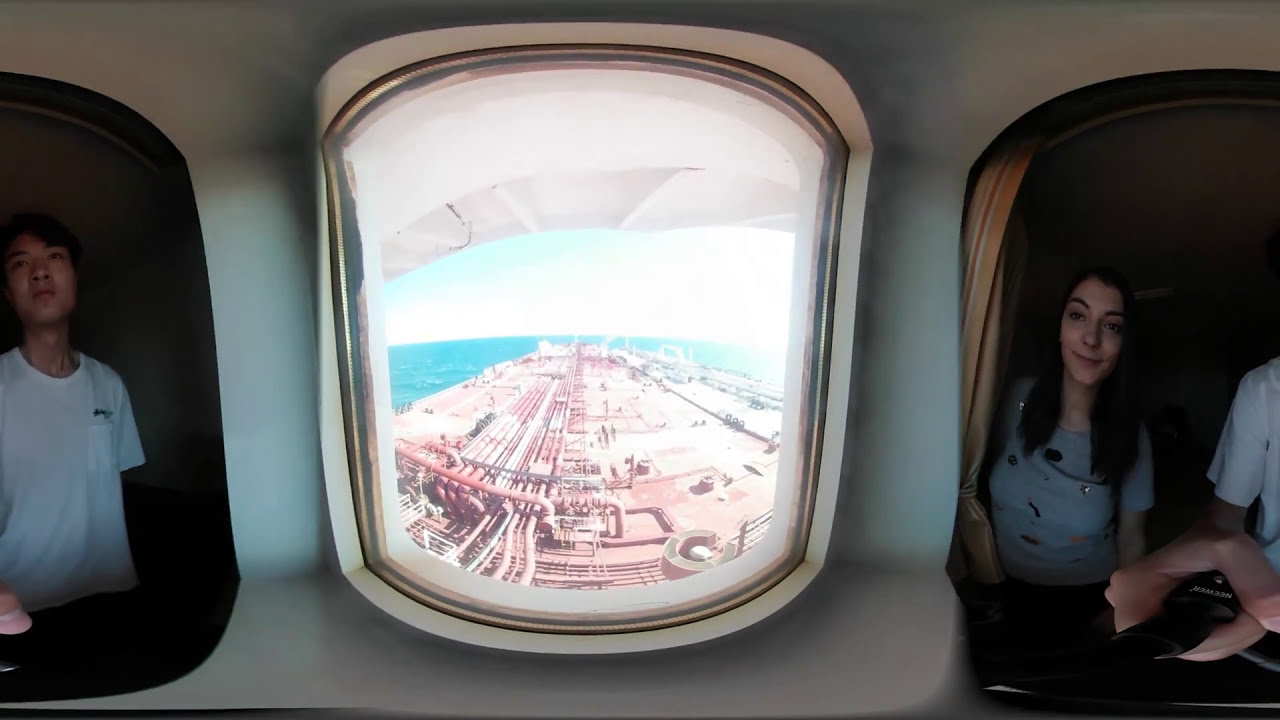In this image, we see a distorted, fish-eye view capturing a group of people inside a room or compartment. They are gazing out of a long, rectangular window framed in white. Outside, the window reveals an expansive body of clear, blue water with a bright blue sky above, situating us on what appears to be a large, industrial vessel—possibly an oil tanker or cargo ship. The exterior scene is filled with metal pipelines and steel structures, indicating a highly industrial environment.

On the right side of the image, there is a woman with long, straight black hair, wearing a gray shirt, who seems to be smiling as she looks out the window. To her left stands a man, possibly of Asian descent, with short dark hair and a white t-shirt, appearing to gaze upwards. Their figure appears somewhat distorted by the fish-eye effect, causing parts of their image to seem repeated or stretched across the frame.

The overall image combines elements of an industrial maritime setting with the personal touch of the individuals inside, looking out into the vast, serene sea and sky.